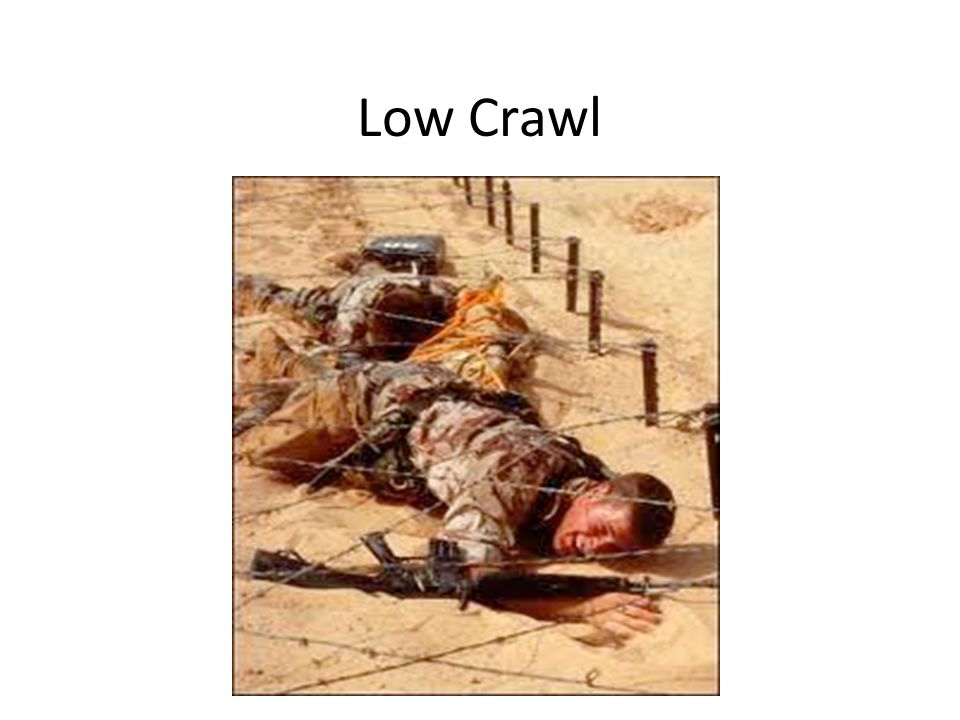In this photograph, titled "Low Crawl" in bold black font above the image, two men in military camouflage are depicted undergoing intense training exercises in a desert-like environment. The soldiers, identifiable by their very short hair, are shown crawling on their stomachs beneath barbed wire that is secured a few inches above the ground by stakes. In the foreground, the more visible soldier grips a rifle by the edge, his face a mixture of concern, concentration, and stress. Although the second man in the background remains partially obscured, his position and posture indicate he is also navigating the course, dragging equipment behind him. Both soldiers wear belts laden with various pouches and military gear, contributing to the sense of a rigorous and demanding training scenario. The image, slightly blurry, evokes a sense of the strenuous physical and mental challenges faced during basic training.